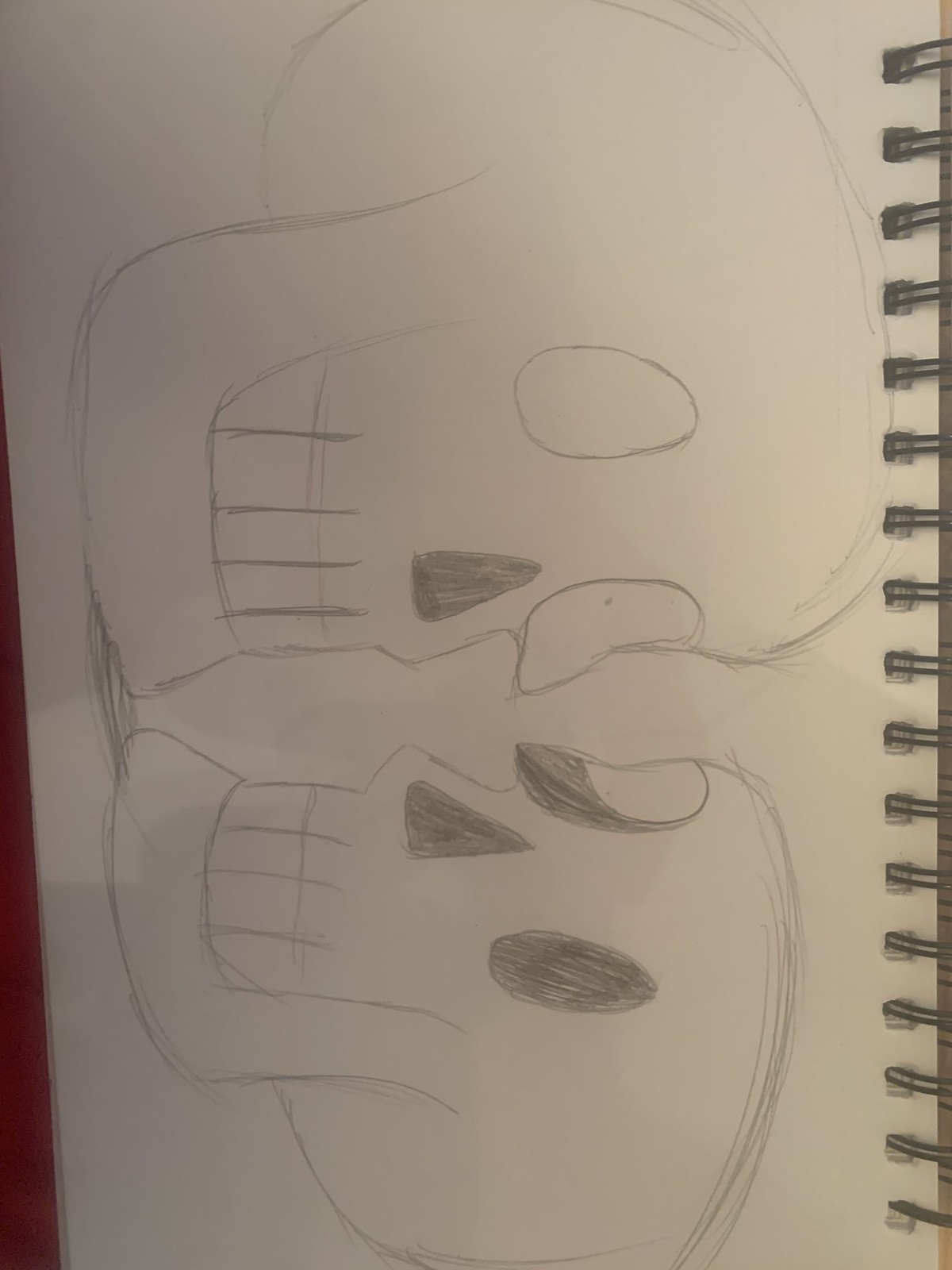A well-used sketchbook lies open, its pages revealing intricately detailed pencil drawings of skeletons. The sketchbook is bound with a metal ring on the right-hand side, through a series of evenly spaced holes. Dominating the page are three skeletons, positioned distinctly at the top, middle, and bottom. Each skeletal figure is expertly rendered with hollowed white eye sockets and dark, shadowy noses, giving them a haunting appearance. The teeth, drawn as large squares, add a stark precision to the otherwise fluid sketches. Beneath the skeletal figures, the fur is depicted as hollowed and textured, created with meticulous pencil strokes. The bottom skeleton's right eye socket stands out with a slightly white shading, contrasting the predominantly dark hues that make up the rest of the illustration.